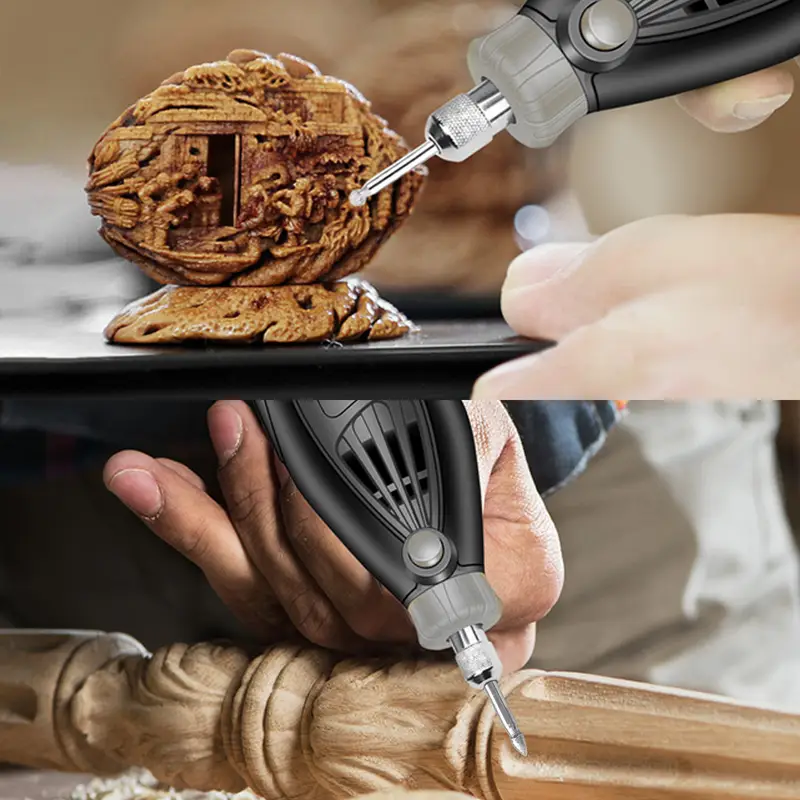The image is a composite photograph showcasing the intricate capabilities of a fine-tipped Dremel-style tool for woodworking. The top half captures a close-up of hands meticulously carving a highly detailed miniature walnut, featuring delicate figures that suggest a scene. The tool's very fine tip is visible, emphasizing its precision for intricate designs. The bottom half shows a continuation of woodworking on a larger scale, with hands using the same tool to refine fluting on a table or chair leg. The leg, already carved in an acanthus leaf style and lathed, is being detailed further, highlighting the tool's versatility for both small and large projects. Set against a backdrop of realistic wood dust, the composite image seems to serve as an advertisement for this advanced fine woodworking tool.